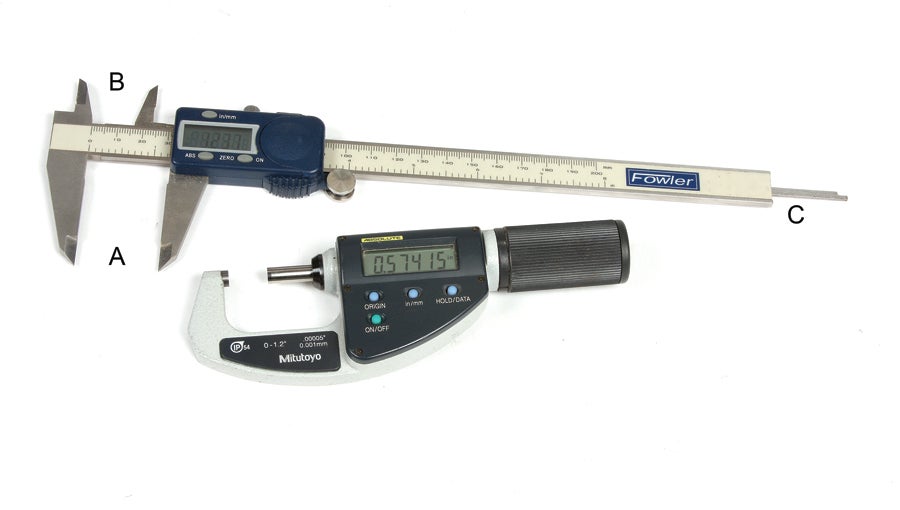This horizontal image features two precision engineering tools, both key instruments for measuring distances with high accuracy. The top tool is a Fowler digital caliper, characterized by its long, slender form and dual sets of arms that extend perpendicularly from the main body. The upper arms, equipped with teeth, are designed to measure the inside dimensions of objects, such as the diameter of cylindrical parts. The lower arms, with straight, pointed edges, measure the outside dimensions. This device features a movable center section with a small window displaying measurements digitally, enabling precise readings as it slides along the integrated ruler.

The bottom tool is a more compact, handheld instrument from the brand MITUTOYO, often used to grasp small objects or likely measure specific forces. It resembles a pair of pliers, with a digital display to the right and a black adjustment knob below. This knob allows users to finely adjust the distance between its two prongs, making it suitable for detailed and precise measurements.